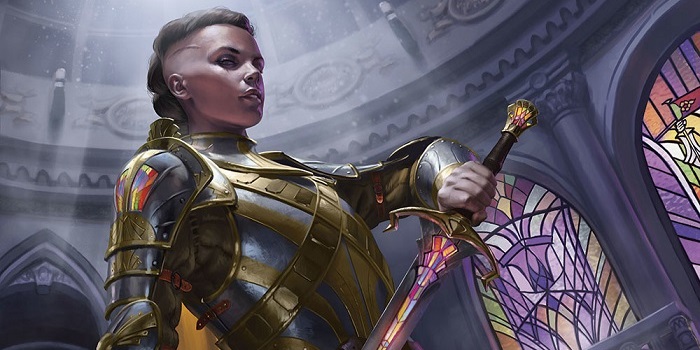The image depicts an animated illustration of a formidable female warrior, potentially a character from a video game or movie. She stands resolute in silver and gold-plated armor. Her distinctive hairstyle features dark brown hair styled into a ponytail, with the sides of her head shaved, revealing a prominent scar on the right side, and a vein bulging, highlighting her determined and aggressive demeanor. She is in the process of drawing a large sword that glows with intricate stained glass-like embellishments on its black and gold hilt, and has a blade with colorful etched designs. Behind her, the Sun shines brightly from the top left corner, illuminating the scene. The background suggests the interior of a grand castle or church, characterized by vibrant stained glass windows of various hues like purple, green, yellow, and orange, and supported by imposing black columns and archways reaching upward, framing the warrior in a heroic and majestic light.